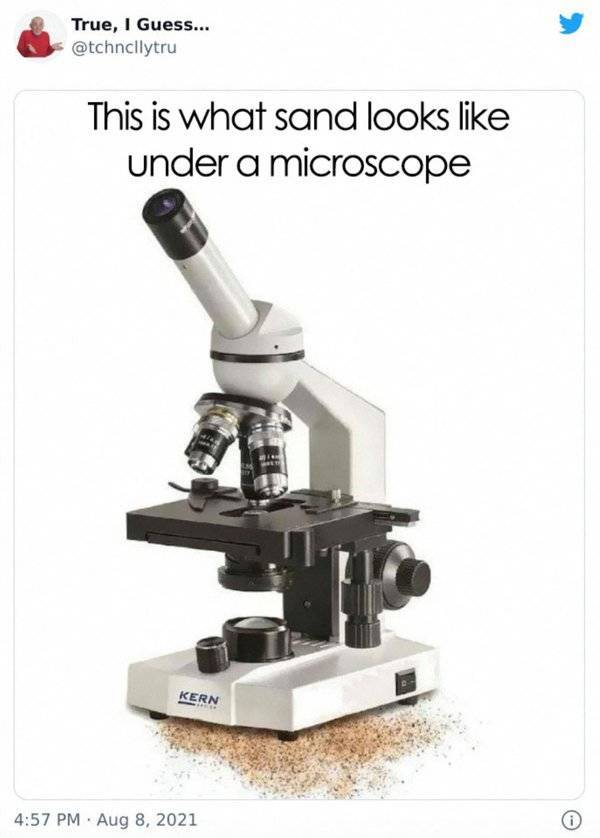This image, a color photograph in portrait orientation, features a white microscope positioned slightly on a small amount of beige and gray sand particles, set against a predominantly white background. The microscope, a product by Kern, is detailed with three lenses, a black base, a bicurved arm, and an eyepiece extension with a black lens. The photograph is integrated into a social media post, framed by a rectangular gray outline. At the top of the post, in black text, reads, "This is what sand looks like under a microscope." Above this heading is the social media user's information, featuring an icon of an older man with his hands raised in a shrug, accompanied by the text "true, I guess..." and the handle "@TCHNCLLYTRU" (Technically True). The upper right corner bears the blue Twitter bird symbol, indicating the platform. At the bottom of the image, a timestamp notes "4:57 p.m., August 8, 2001," cementing the moment this content was shared. The style of the image combines photographic realism with social media typography, presenting scientific equipment in an accessible digital format.